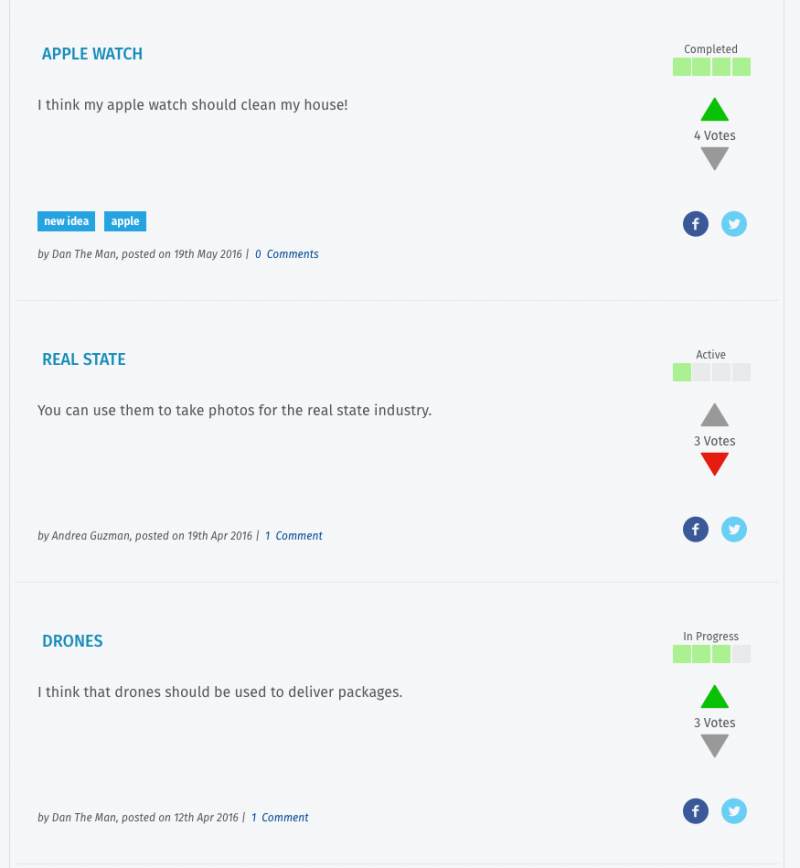The image displays a website interface with a clear blue-themed background. On the left side, there are several entries related to tech ideas and innovations:

1. At the top, in blue text, "Apple Watch" is prominently displayed. Below, a humorous suggestion reads, "I think my Apple Watch should clean my house." This idea is marked as "completed," supported by four green vote boxes, indicated by four votes. A green arrow points up, showing approval, while a gray arrow underneath shows no dissent.

2. To the left, another entry is labeled "New Idea" in a blue box, adjacent to the topic "Apple," also in a blue box. This entry, posted by Dan the Moon on May 19th, 2016, has garnered nine comments.

3. Further down, another entry under the category "Real Estate" in blue suggests using a certain technology to take photos for the real estate industry. This idea is marked as "active" with a green label and has received three votes. A red triangle points down, indicating some level of disapproval beneath a gray triangle indicating neutrality or no votes.

4. An idea under the category "Drones," also in blue, proposes using drones to deliver packages. This suggestion is labeled "in progress" and is accompanied by three green progress bars. Similarly, it has a green triangle going up and a gray triangle going down, reflecting mixed feedback. This entry was posted by Dan the Moon on April 12th, 2016.

At the bottom corner, icons for Facebook and Twitter are displayed, suggesting options for sharing the content on social media platforms.